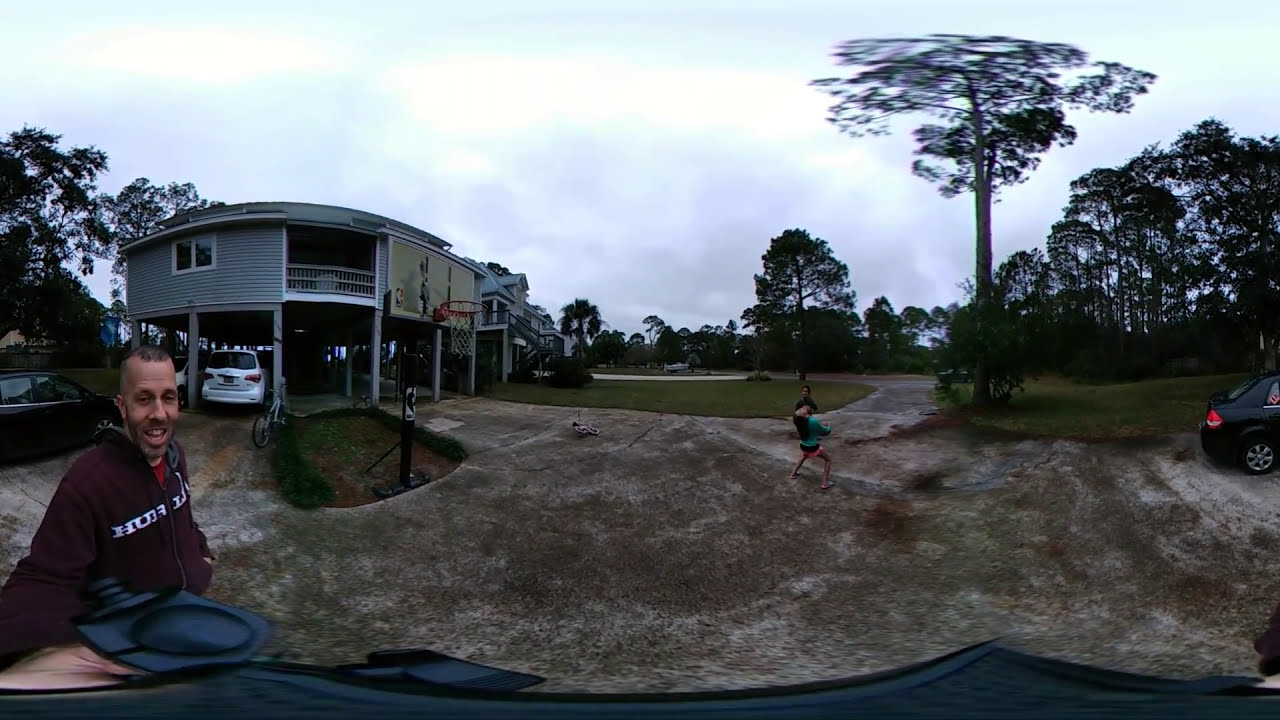This panoramic photograph captures an outdoor scene in front of a house elevated on stilts. The house, featuring a grey exterior with tan trim, stands prominently with two cars parked beneath it—one white and the other black, the latter partially cropped on the left and extending into the right side of the image. Beside one of the stilts, a bicycle is visible, and a basketball goal is attached to the side of the house, with an orange rim adding a pop of color. The overcast sky casts a diffused light, emphasizing the absence of direct sunlight.

In the foreground, a man with caramel-colored skin, likely South Asian in ethnicity, is capturing the photo. He smiles at the camera, dressed in a dark purple hoodie. To his left, two children are seen playing joyfully in the long concrete driveway, which leads out to a small lawn and a grove of tall pine trees in the background. A dirt driveway extends beside the concrete one, showing varied textures of brown and off-white amidst the greenery. The trees and other elements transition smoothly but are slightly blurred, adding to the panoramic feel. Additionally, another man in the background, wearing a hoodie with some indistinguishable text, adds to the casual, bustling atmosphere of this everyday moment captured outdoors.